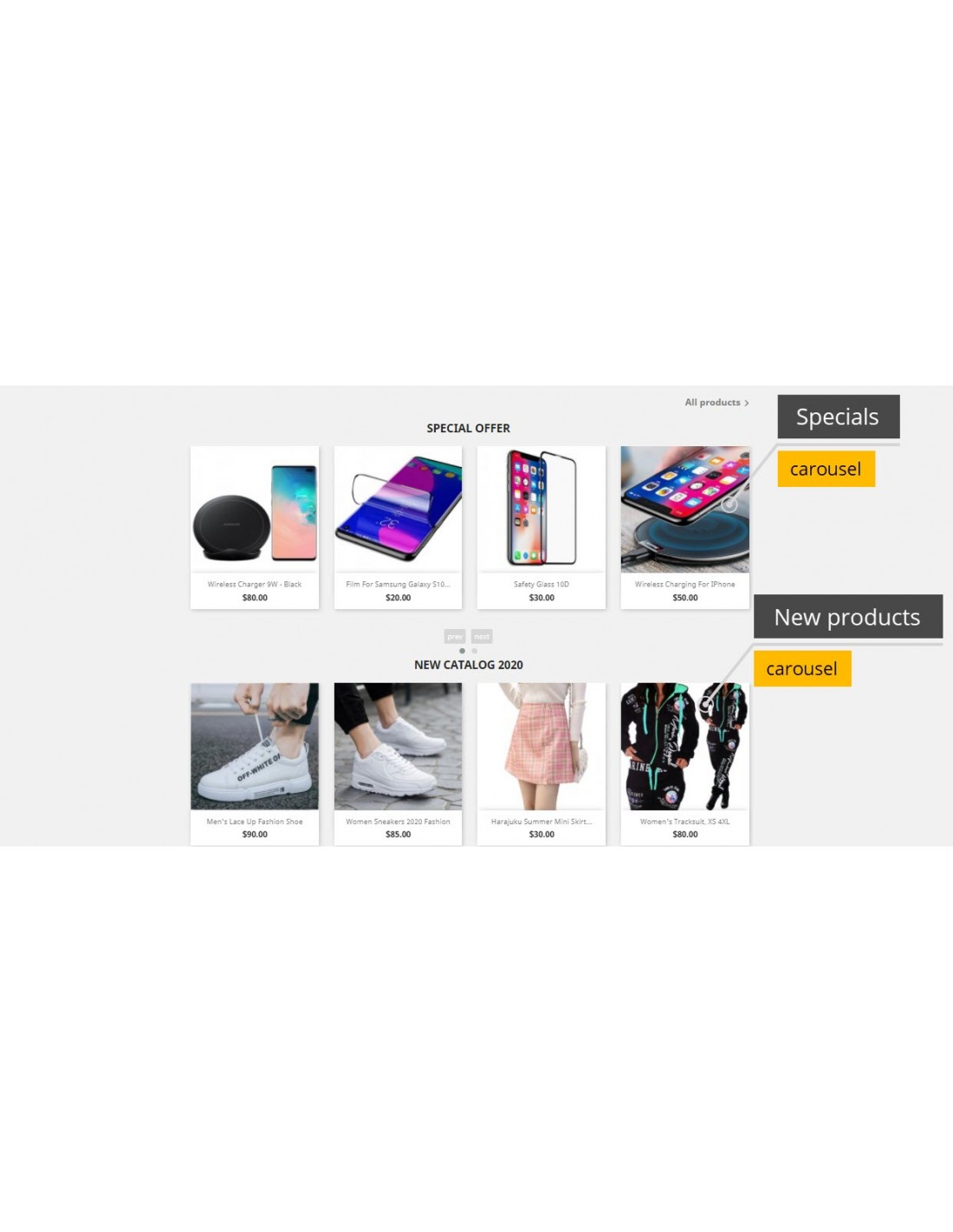The image displays a digital screen featuring special offers. The top section showcases various phone accessories, while the bottom section highlights clothing products. Due to the small text, the descriptions are difficult to read. Specifically, the phone accessories include a screen protector, a shield cover, and a charger, all seemingly designed for iPhones. The clothing items featured are a pair of white sneakers, a pink plaid skirt paired with a long white sleeve shirt, and a black jumpsuit with white and green accents. The interface utilizes a black-and-white theme for the special offers and a combination of orange and black for the carousel. Users can navigate through the items, highlighting their choice and selecting it for more details.